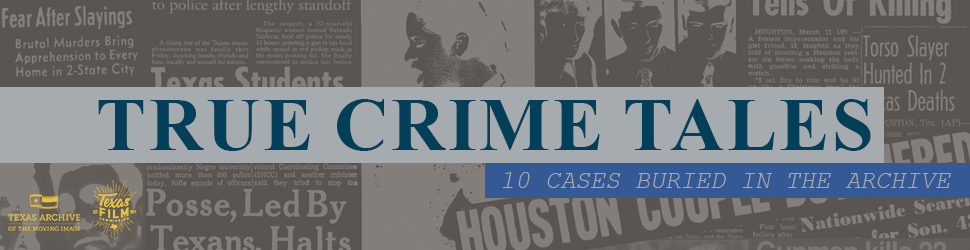The image is a narrow, horizontal banner with a striking design that prominently features text and a background of inverted newspaper clippings. The headline, "True Crime Tales," stands out in dark blue against an off-white background, while the subheading, "Ten Cases Buried in the Archive," is displayed in white lettering on a lighter blue strip. The intriguing background consists of various overlays of negative photo images where the white has turned black and the black has turned white. These newspaper clippings feature chilling headlines and phrases such as "Fear of Slayings," "Brutal Murders Bring Apprehension to Every Home in Two-State City," "Texas Students," "Posse Led by Texans Halts," "Houston," and "Nationwide Search." The unsettling collage of articles, some barely legible, evokes the mystery and horror associated with true crime stories.